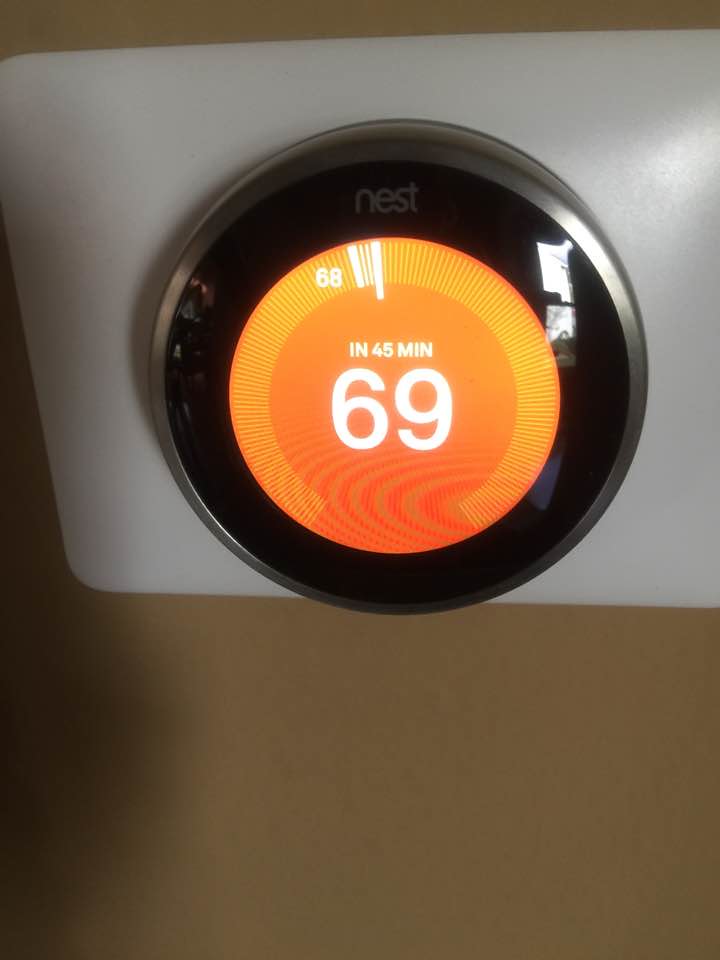This photograph captures a Nest thermostat control unit mounted on an indoor wall. The prominent source of light illuminating the scene is a nearby window, its reflection discernible on the right side of the dial. This reflection highlights the sleek white plastic of the control unit, the silver trim around the dial, and the glassy surface of the central black digital display. The wall behind the unit is painted in a warm beige or sand hue.

The thermostat itself is a sophisticated square device made of white plastic, featuring a central circular dial with a silver trim. Within the dial, a black digital display is set, covered by a glass front. The display is primarily black, showcasing a central gauge with orange detailing and yellow lines demarcating each degree of temperature. At the very top of the black circle, the brand name "nest" is subtly inscribed in a grey font with a lowercase "n."

The displayed temperature reads 69 degrees, accompanied by a note that says "in 45 minutes," likely indicating the expected time for the temperature to reach the desired setting. On the outer edge of the display, the temperature increment of 68 degrees is marked with lit white lines, providing a clear, visual reference point.